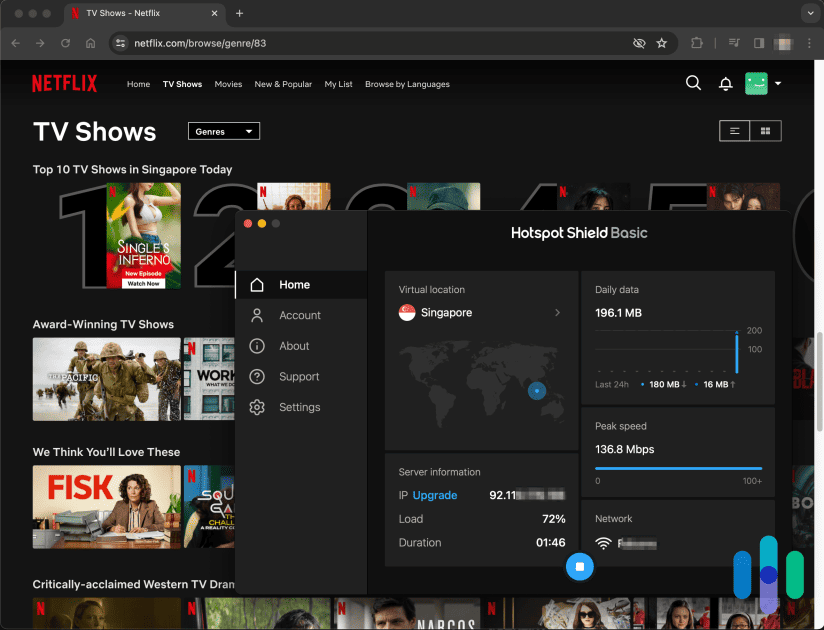Screenshot of the Netflix Home Page with Various Highlighted Content

The given image is a screenshot of the Netflix website. The primary background color is black, creating a sleek and modern interface. At the top of the screen in the browser tab, the familiar red "N" logo for Netflix is visible, with the tab title displaying "TV Shows - Netflix" in white. The URL indicates the page is located at "netflix.com/browse/genre/83".

On the left side, in bold red and all capital letters, the word "NETFLIX" appears prominently. To the right of the Netflix logo, there are six navigation categories: "Home," "TV Shows," "Movies," "New & Popular," "My List," and "Browse by Languages." The category "TV Shows" is currently highlighted, suggesting this section is active.

Directly beneath the Netflix logo, "TV Shows" is written in white font. Next to it, there is a drop-down box labeled "Genres," which allows users to filter TV show categories.

Below this primary navigation, a section titled "Top 10 TV Shows in Singapore Today" lists popular shows. The top spot is occupied by "Singles Inferno," although the following ranks (2 through 5) are not visible in the screenshot. Beneath this list, a section labeled "Award-Winning TV Shows" is partially displayed, with only "Pacific" visible as part of a title.

Further down, there's a section named "We Think You'll Love These," showcasing "Fisk" and "Squid Games." Below this, a category titled "Critically Acclaimed Western TV Dramas" is mentioned, although the associated images are not fully visible.

Additionally, there is a black overlay box at the top of the website showing a white text header: "Hotspot Shield Basic." This box includes five categories on the left: "Home," "Account," "About," "Support," and "Settings." It also displays a virtual location set to Singapore, with daily data usage of "196.1 MB," and other details related to server information, including peak speed and network status.